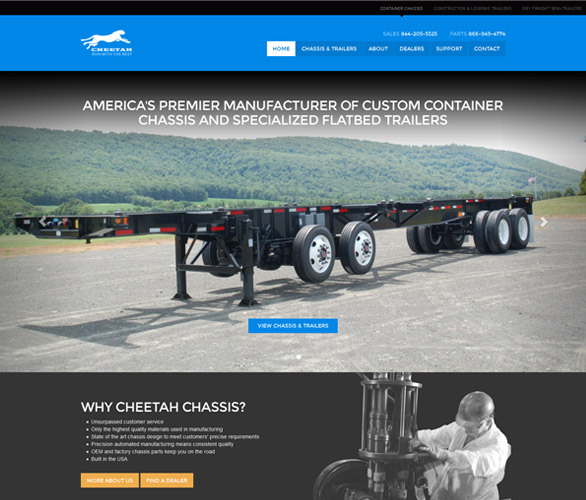The image is a screenshot of a website with a detailed layout. At the very top is a black bar, followed by a blue banner. Dominating the banner is an image of a white cheetah in mid-leap with the word "Cheetah" written beneath it, accompanied by some unreadable text. On the middle and right side of the banner, there are two phone numbers, likely labeled "Sales" and "Parts."

Below the banner are the following tabs listed from left to right: "Home" (which is currently selected), "Chassis and Trailers," "About," "Dealers," "Support," and "Contact."

The main section of the website features a large photograph showcasing an outdoor scene with rolling hills and trees in the background. The foreground shows a flatbed trailer on a paved surface, missing the cab that would typically pull it. This trailer has two sets of wheels—four in the front and eight in the back—with red and white reflective tape along its sides. The trailer is supported by props.

Beneath the main photo is a blue bar with the text "View Chassis and Trailers." Directly under this is a black bar that features an image of a man in a white coat and hard hat, working at an unidentified machine. To the left of this image, the text "Why Cheetah Chassis" is displayed above an unreadable bulleted list. At the bottom, there are two yellow buttons labeled "More About Us" and "Find a Dealer."